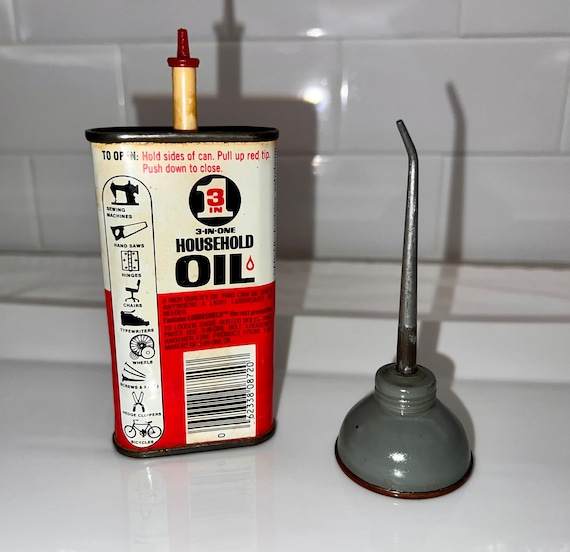In an indoor setting, the photograph showcases two oil cans placed on a shiny, white tiled surface. The background features a matching white tiled wall, creating a clean and cohesive look. On the left, there is a tall, cylindrical can, black and red in color with a white upper section. The can is labeled "3-in-1 Household Oil" and displays various instructions and a barcode. The can also features illustrations of items such as a sewing machine, saw, hinges, chairs, and bicycles, indicating its versatile applications. At the top of this can is a cylindrical nozzle with a small, red dropper tip, designed for precise oil application.

Adjacent to this oil can, on the right, is a grey funnel with a rounded base that transitions into a long metal nozzle. The funnel appears sleek and shiny, complementing the polished surface it rests on. Together, these items give the impression of products typically found in a hardware store, essential for various household and repair tasks.